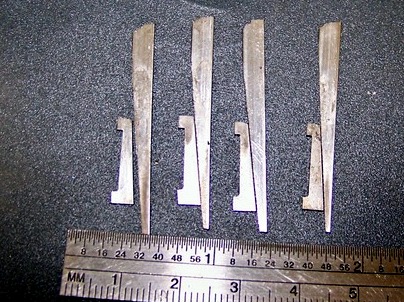The color photograph features a diagonally positioned metal ruler along the bottom edge, extending from left to right, and measuring up to approximately seven inches. The ruler slightly descends to the right and displays a reflection of a light source at its center. Positioned against a dark grey, short-pile carpet background, there are four pairs of metallic pieces above the ruler. Each pair consists of a long, tapered piece, resembling a propeller blade, and a shorter, back-to-front C-shaped piece with short projections. Despite slight color variations, all pieces share a gold, shimmery appearance.